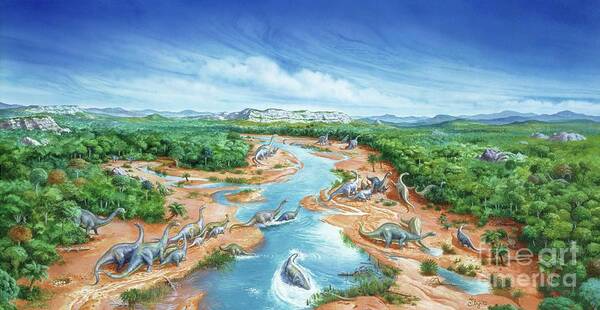This vibrant painting depicts a prehistoric scene from the Pleistocene era, teeming with a variety of dinosaurs. Dominating the composition is a river that winds through the center, curving slightly to the left. On either side of the river, the landscape transitions from sandy riverbanks to lush, bright green jungles. This dense foliage, which almost resembles a forest, is scattered with numerous long-necked dinosaurs, likely brontosauruses, crossing the river at a narrow point. These dinosaurs, portrayed in shiny gray hues, are joined by other species, including smaller dinosaurs, in various colors such as blue, dark blue, and green. 

In the background, majestic, rocky gray mountains rise against a beautiful expanse of blue sky, dotted with white clouds. The scene is highly detailed, with meticulous attention to the bright colors—greens, tans, and blues—that make the ancient landscape come alive. The bottom right corner of the painting contains a watermark reading "Fine Art America," grounding this artwork in its authentic artistry.